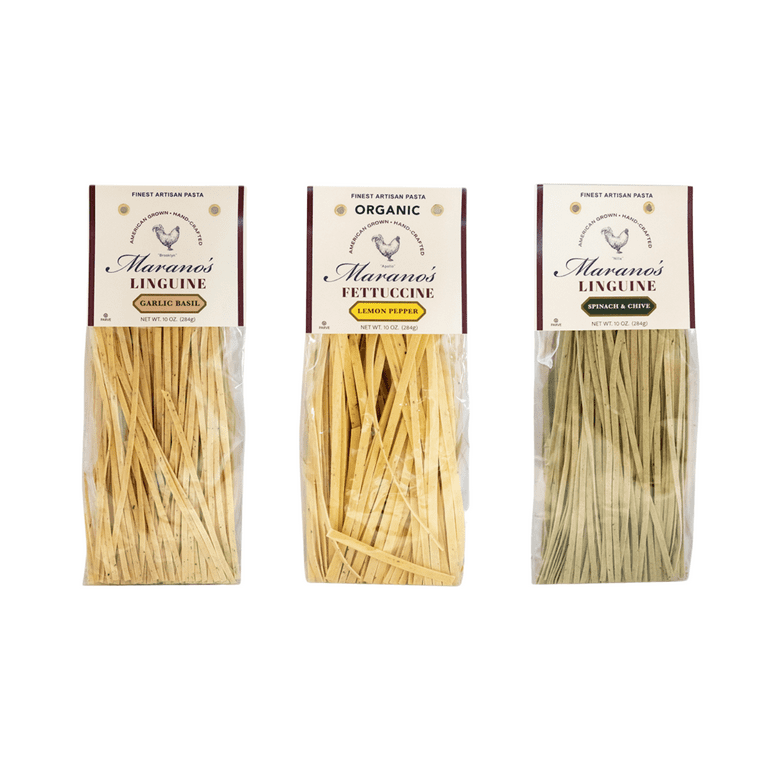The image features three packages of Mariano's artisanal pasta displayed vertically against a white background. Each package consists of clear cellophane-wrapped pasta with a cardboard label. The packaging allows visibility of the pasta inside and includes detailed labels with a prominent rooster logo and the net weight indicated.

The first package on the left showcases Mariano's Linguine Garlic Basil with an off-white label and brown text. The pasta inside is a darker yellow hue, suggesting a hearty flavor mix of garlic and basil.

In the middle, there is the organic option, labeled as Mariano's Fettuccine Lemon Pepper. This package features the words "lemon pepper" in bold yellow letters on the off-white label, and the pasta inside is a brighter, light-colored fettuccine, indicating the zesty lemon and pepper blend.

The package on the right contains Mariano's Linguine Spinach and Chive. The label displays green text highlighting the spinach and chive flavor, and the pasta inside has a light green tint, reflecting its fresh, herbaceous ingredients.

Overall, the clear and consistent branding, combined with the transparent packaging, showcases the varied colors and artisanal nature of these handmade-looking pastas.